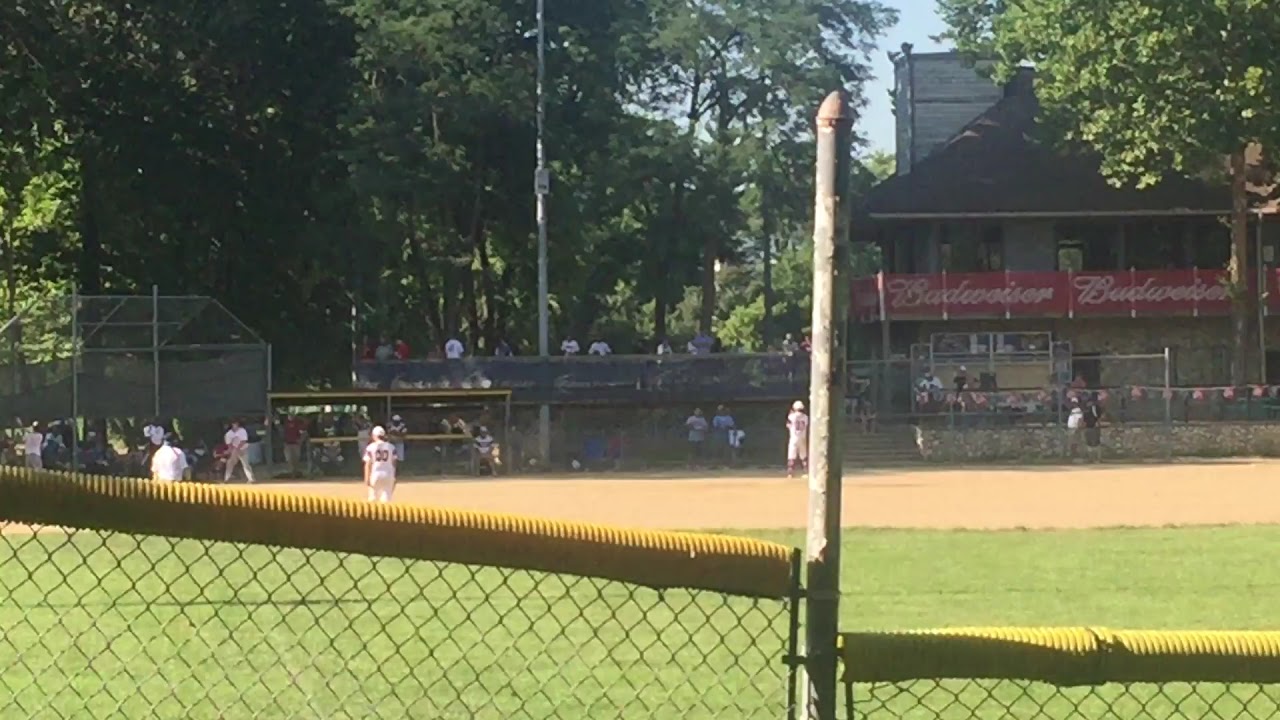The image captures a lively baseball game being played on a sunny day. Taken from the perspective behind the right-field fence, the scene is set on a small baseball field, possibly belonging to a high school, amateur league, or small college. The players are in their positions, with the pitcher poised to throw the ball and the batter ready to hit. The players are dressed in white uniforms with numbers on their backs. In the background, a building with a large red Budweiser sign across its second level stands prominently, suggesting it might be a concession stand selling beer, nachos, or pretzels for the spectators. The stands behind the left portion of the field are filled with fans enjoying the game. The surrounding trees are in full bloom, indicating that the game is taking place in the summer. Overall, the vibrant atmosphere and presence of spectators suggest that everyone is enjoying the sunny day and the excitement of the baseball game.